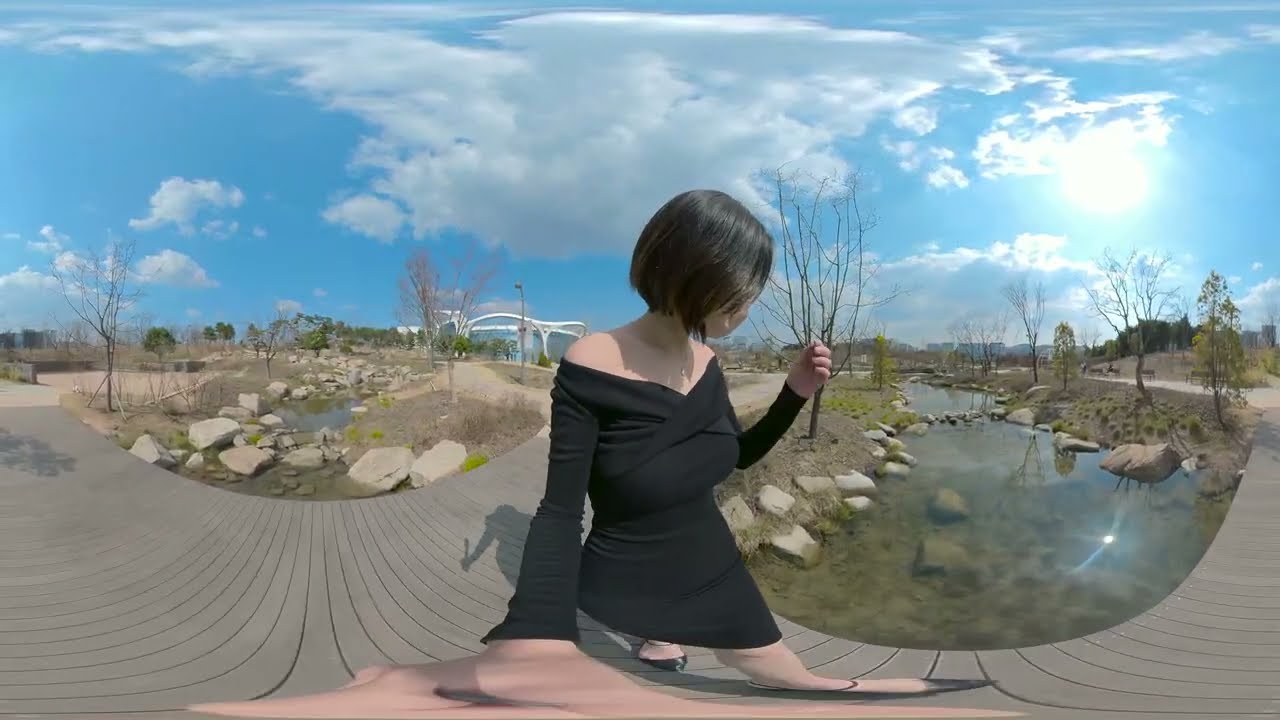The image showcases a woman standing front and center, with straight, black hair cut to her chin, and she is wearing a form-fitting, dressy black outfit that could either be a dress or a stretch shirt. She has on sharp black shoes and is standing on a boardwalk that appears to be gray and made of a plasticine or Trex material. The boardwalk goes in multiple directions, forming a circular pattern.

In the background, there are two shallow ponds adorned with rocks, alongside a small brook or stream. Around these water features are numerous trees; some have leaves while others are bare. Further in the distance, you can also make out more trees and a white, curvy-topped building with plenty of glass. The sky is a vibrant blue, punctuated by puffy white clouds and an abundance of sunlight streaming through, creating a serene and picturesque scene.